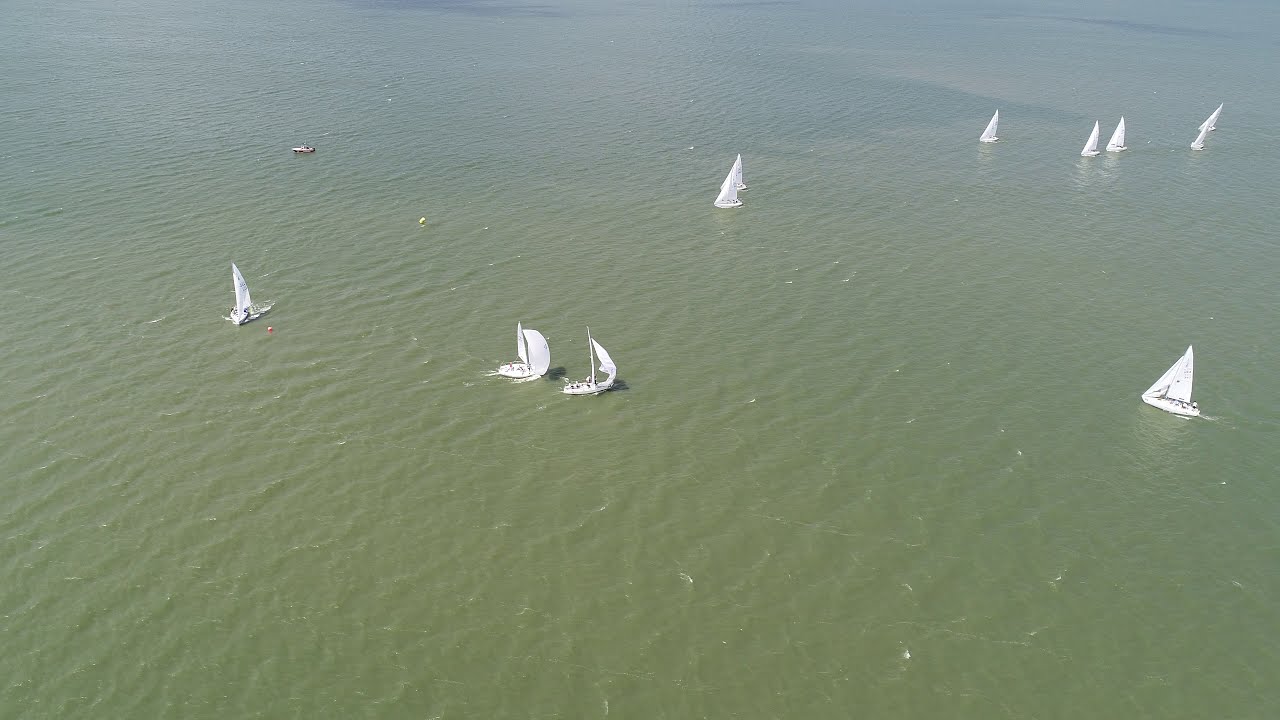This aerial photograph captures a large, greenish and somewhat muddy body of water. The scene is enveloped in a hazy, overcast atmosphere, suggesting it's not a bright and sunny day. Spread across the water are 11 white sailboats, all with white sails, arranged in a distinct pattern. Some sailboats are heading left while others, turning around a buoy, are moving back to the right, seemingly propelled by a stronger wind. Additionally, a large, flat, brown boat can be seen towards the upper left corner. In the water, fish are visible near the surface, contributing to the dynamic nature of the scene.